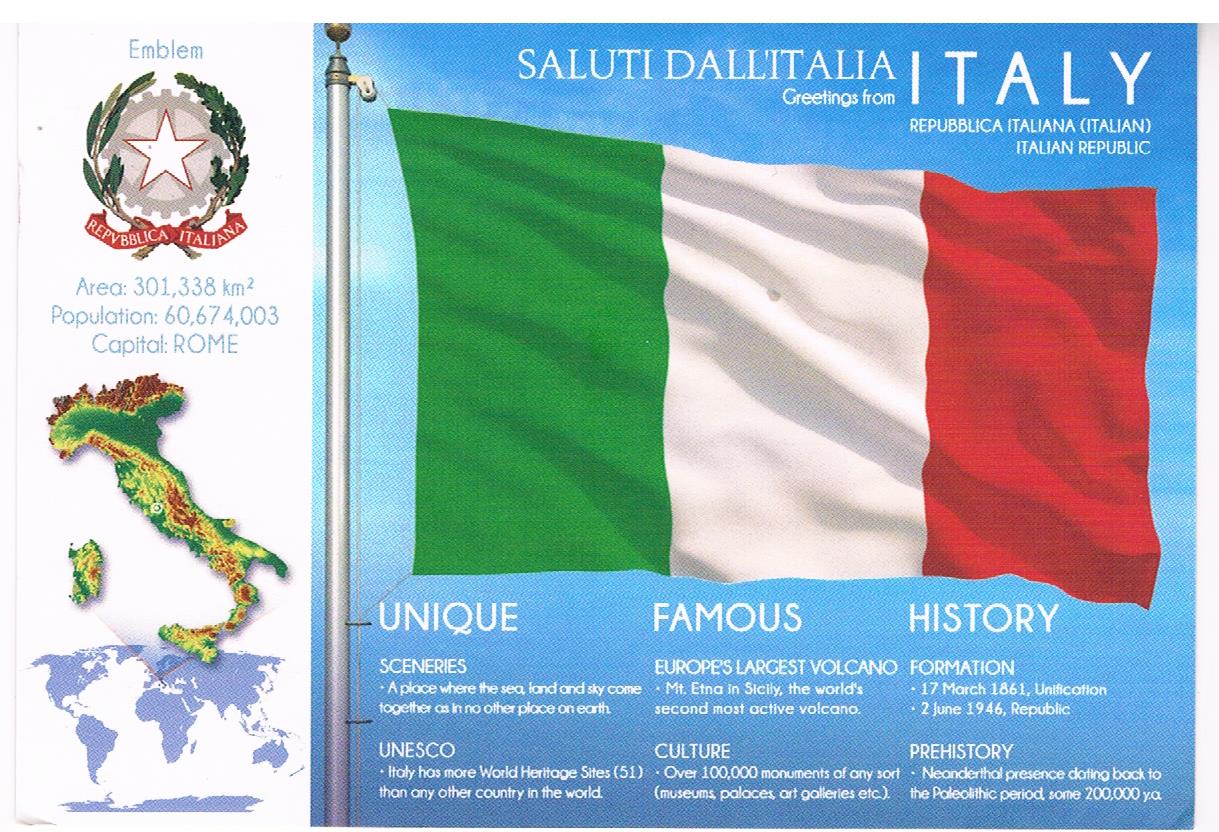This image appears to be a detailed poster or card about Italy. The right-hand side features a dominant "Greetings from Italy" section set against a blue sky background. Central to this area is the Italian flag, waving majestically on a flagpole, divided into three vertical sections—green on the left, white in the middle, and red on the right. This section is larger and emphasizes Italy’s unique scenery, famous landmarks, cultural richness, historical significance, and prehistory, with all the descriptive lettering in white.

On the left-hand side, a smaller portion of the poster showcases Italy's emblem, which consists of a white star placed at the top left corner, encircled by a green wreath resembling an open semicircle at the top, and a red banner at the bottom. Below the emblem, there's detailed information including a map of Italy, which appears green, yellow, and brown, resembling the shape of a boot. The map also identifies Italy's population as 60,674,003 and lists Rome as its capital. Additionally, there’s another map that positions Italy within the global context. Most of the text and information in this section is written in Italian, adding to the authentic feel of the poster.